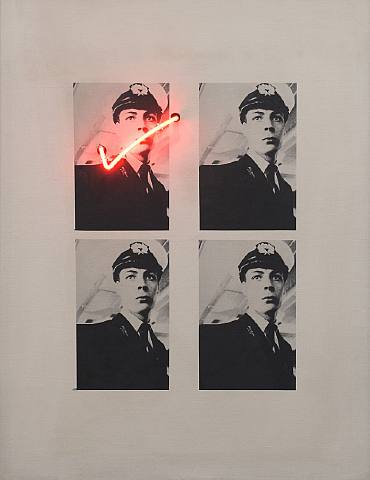The graphic artwork features a repetitive motif of a naval officer, positioned in a 2x2 grid pattern against a background that transitions between dark brown and light gray. The officer, depicted in black and white, is wearing a formal naval uniform complete with a white hat adorned with an insignia, a black jacket, a white collared shirt, a black tie, and brass emblems on the collar. Each image portrays the officer looking solemnly at the camera without a smile, his head turned slightly. Notably, the top left image is distinct from the others due to a striking red neon checkmark that overlays and extends across the officer's face and uniform, creating a stark contrast. The other three images remain uniform and identical, contributing to the collage's cohesive yet punctuated visual narrative.